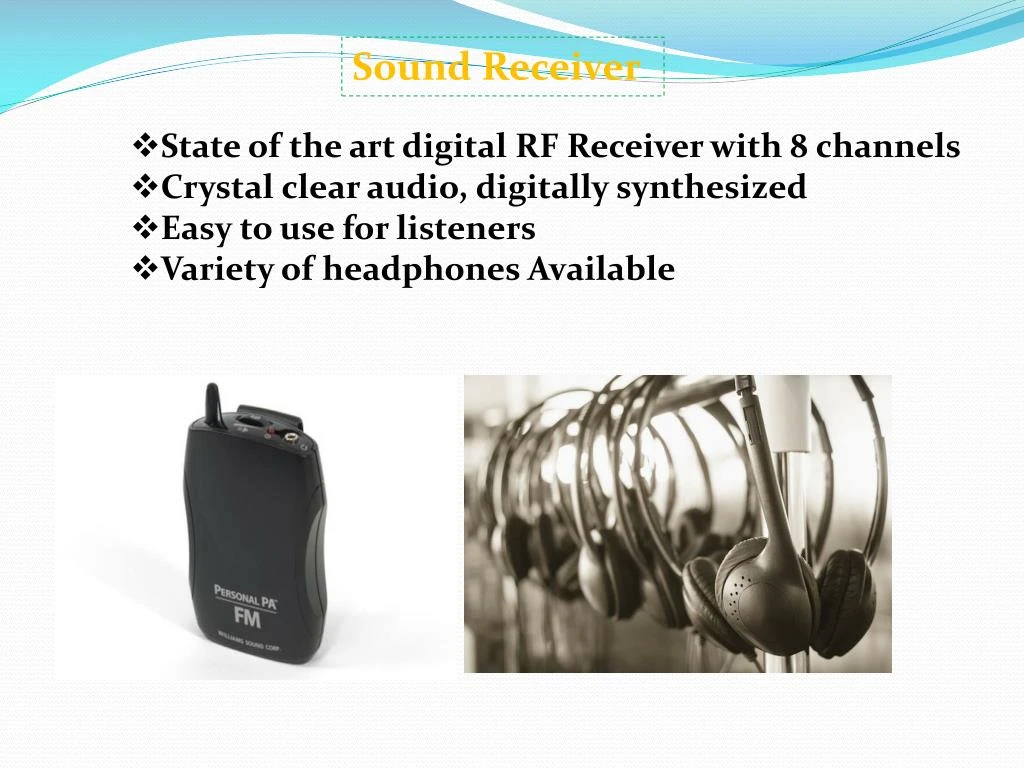The image appears to be a slide from a presentation featuring a product called a sound receiver. The slide has a blue and white header with wave-like designs at the top, set against a primarily white background. At the top of the slide, within a green dotted box, there is yellow text that reads "sound receiver." Below, there are four bulleted points, each contained in stylized diamond-shaped bullets. The points read: "State-of-the-art digital RF receiver with eight channels," "Crystal-clear audio, digitally synthesized," "Easy to use for listeners," and "Variety of headphones available."

In the main part of the image, two pictures are showcased. On the left, there is a small, black handheld radio receiver with a beveled rectangular design and a small antenna. The device is labeled "Personal PA_FM." On the right, there is a display rack featuring several pairs of old-school headphones with large ear cups and thin headbands, all arranged neatly on a horizontal bar. The overall design of the slide is clean and focused on clearly presenting the features and appearance of the sound receiver and its accessories.